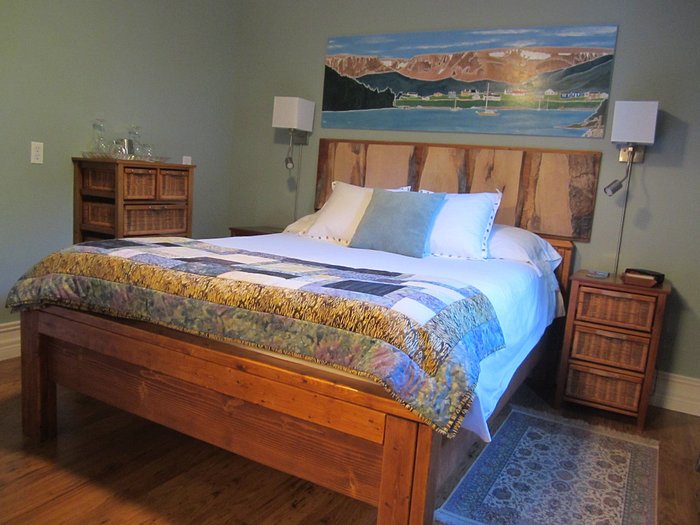The image showcases a cozy bedroom with oak-colored hardwood floors. At the center of the scene is a wooden bed with a substantial headboard and footboard, both crafted in oak but with distinct styles. The bed is adorned with a comforter that has a woodsy design at the bottom and is white on top, complemented by neatly arranged pillows. Flanking the bed are two matching wooden nightstands, each hosting a modern lamp. 

Above the bed hangs a captivating painting depicting a serene landscape: a lake surrounded by snowy mountains and a clear blue sky. The walls are painted green, enhancing the natural theme of the room. On the right nightstand, there is a book placed neatly alongside the lamp. A small carpet lies next to the bed, adding a touch of warmth to the room. 

Situated on the left side of the room is a rustic oak dresser, contributing to the cohesive wood theme. Overall, the room exudes a tranquil and organized atmosphere, perfectly blending modern and rustic elements.